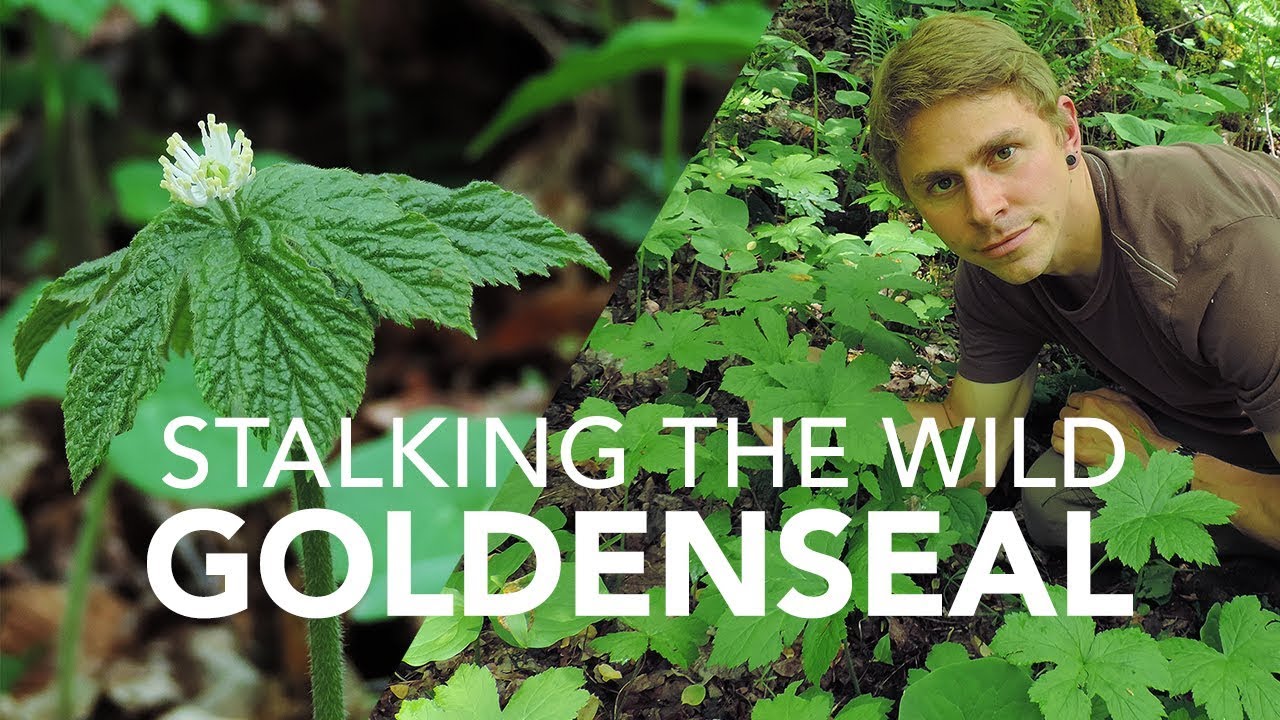The image appears to be an advertisement or an informative picture, created in the style of a video thumbnail. It features two photographs edited together diagonally. On the right side, a man is lying on his stomach, propped up on his elbows, in a lush outdoor setting among greenery, possibly in a wooded area or garden bed. He appears to be in his late 20s or early 30s, with light skin, rosy cheeks, brown eyes, pink lips, and short brown hair feathered to the left. He wears black stud earrings and a brown crewneck t-shirt with white stripes around the collar and shoulders. The man looks directly at the camera with a slight smile. On the left side of the image is a close-up of leaves and possibly a flowering part of a golden seal plant. At the bottom of the image, in white lettering, is the text: "Stalking the Wild Golden Seal."